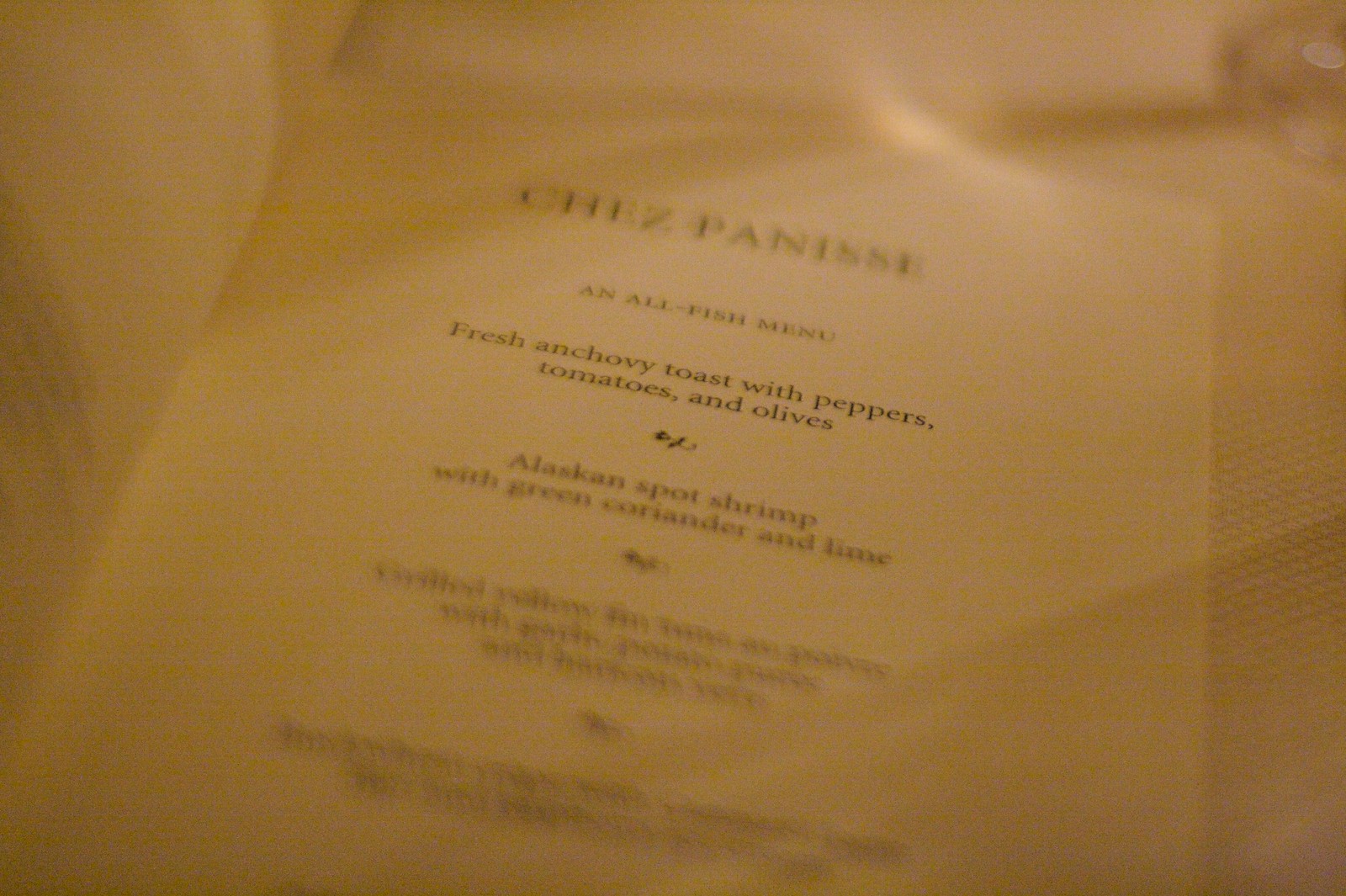This image features a menu page from the upscale restaurant Chez Panisse. The menu is printed on a cream-colored sheet with black ink in a text-style font. Due to the blurry, angled photograph, the clarity diminishes towards the bottom, making it challenging to read the entire content. However, the top of the menu clearly states "Chez Panisse" and "An All Fish Menu." The first two listed dishes are fresh anchovy toast with peppers, tomatoes, and olives, followed by Alaskan spot shrimp with green coriander and lime. The remaining two dishes are unreadable due to the blurriness. The absence of prices implies this establishment serves high-end, gourmet cuisine.